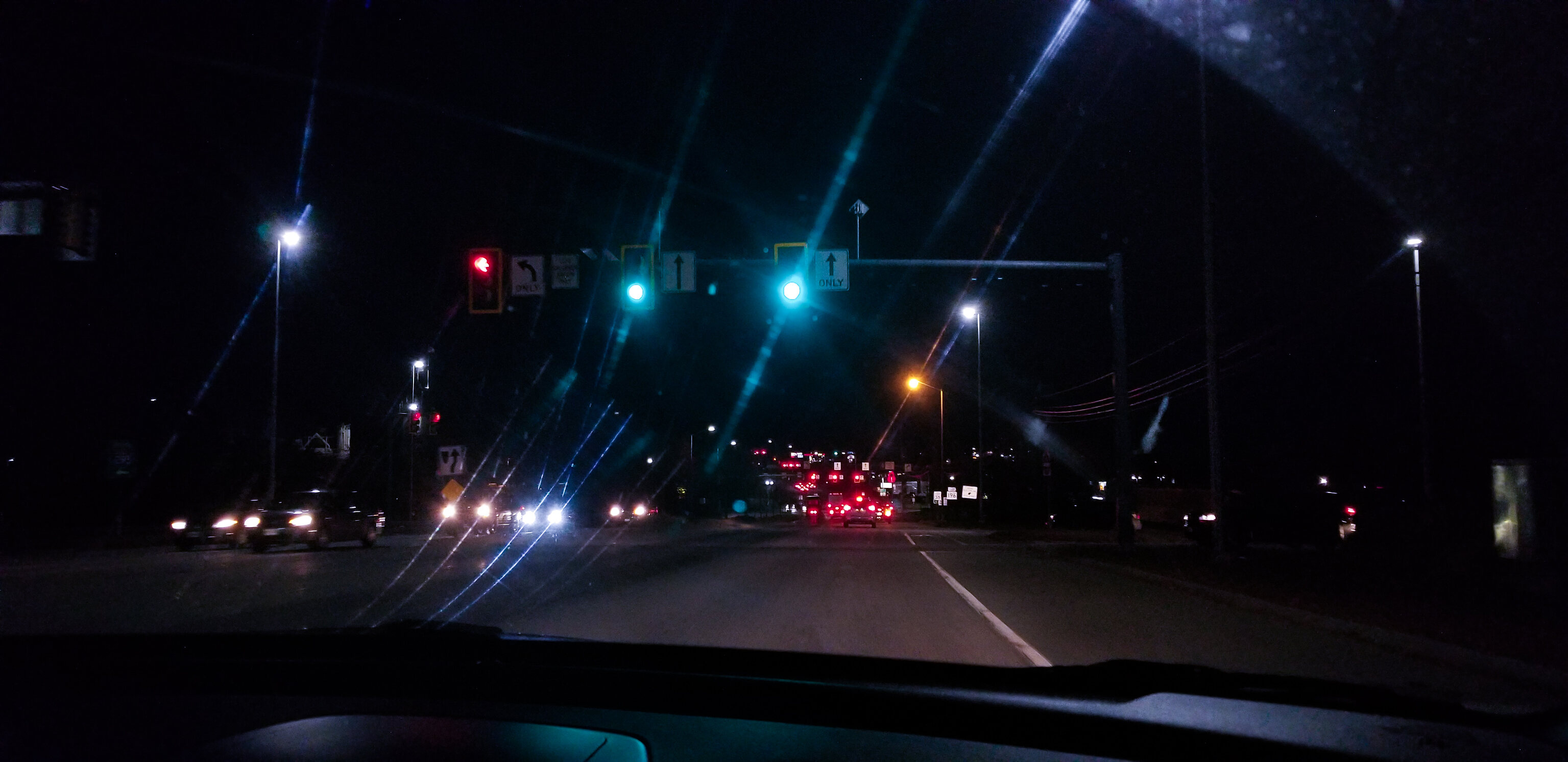The image is a night-time outdoor photograph taken from inside an American car, looking through the front windshield. The scene is of a two-lane street with minimal light, dominated by the dark, black sky. In the center foreground, a vertical streetlight pole features two green traffic lights, each accompanied by rectangular signs with upward-pointing arrows. The illuminated green lights and the signs are clear, though they cast a slight blur and light streak due to the darkness. Up ahead, red taillights from cars in the same lane are visible, creating a trail of light in the distance. To the left, opposing traffic shows several cars with bright headlights heading towards the camera, contributing to light glares on the windshield. The right side of the image is mostly in shadow, save for a single streetlight casting a narrow beam downward. The photograph captures the limited but distinct illumination from various vehicle lights and street fixtures, highlighting the contrast against the almost pitch-dark surroundings.